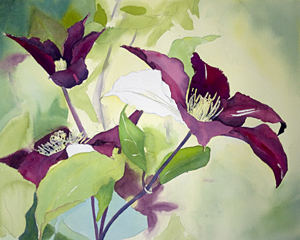The image appears to be an exquisitely detailed painting that resembles a scene straight out of an animated film. It has a delicate, aquarelle-like quality with softly blended colors. The composition predominantly features an abstract field of light green hues, suggesting a lush garden setting. 

In the center and extending to the left side, vibrant plants are depicted in various stages of blooming. The flowers are particularly striking, characterized by their dark purple petals with vibrant yellow centers, creating a beautiful contrast. There are also white flowers interspersed among the purple ones, adding to the rich diversity of the scene.

The overall effect is one of natural beauty and peacefulness, captured in a very small, yet meticulously detailed format. This miniature artwork masterfully conveys the essence of a thriving garden through its use of color and form.